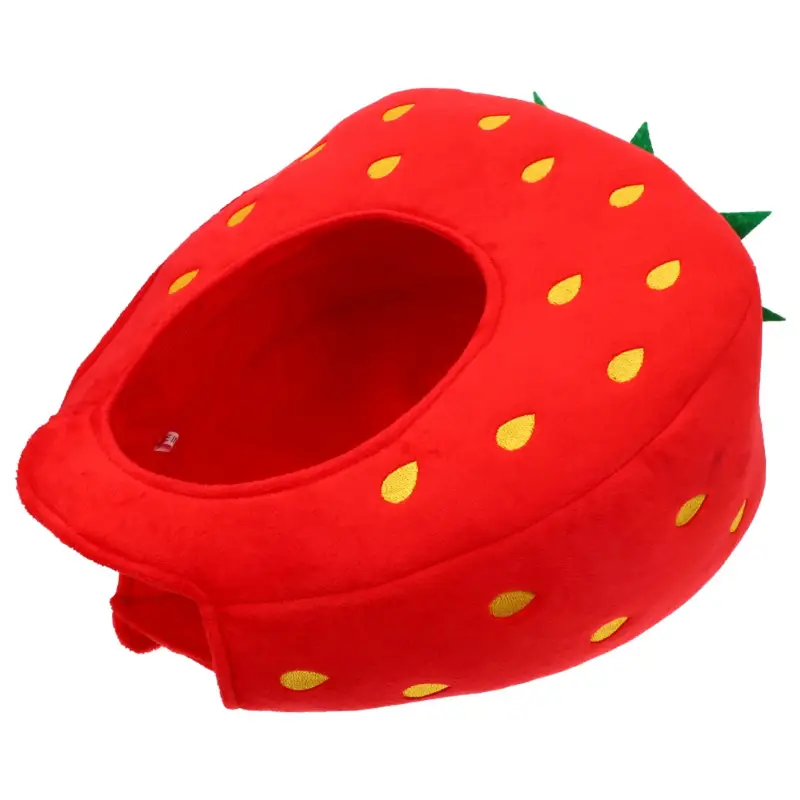This professionally photographed image showcases a large, plush strawberry-shaped headgear or pillow designed to resemble a strawberry costume accessory. The plush item features a vibrant red color with embedded yellow, teardrop-shaped seeds that create subtle indentations on the surface, adding to its realistic texture. At the top of the strawberry, green leaves mimic a crown, making the costume even more lifelike. The item has a central hole, large enough to fit a head, suggesting it can be worn as a novelty headpiece, possibly for Halloween or as a humorous gift. Positioned on a stark white background, a tiny, white, and black tag is visible inside the opening, though its text is undecipherable. This quirky and playful accessory has a commercial appearance, resembling a product that could be found on retail platforms like Amazon.